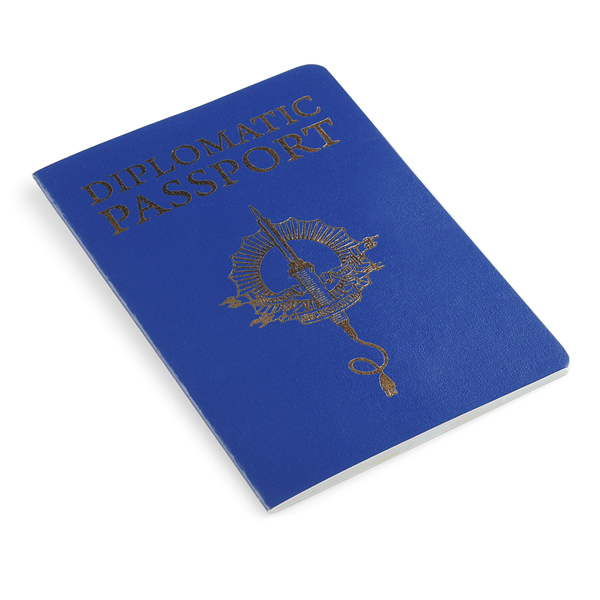The image depicts a blue diplomatic passport cover, likely made of blue leather. At the top, the embossed gold lettering reads "Diplomatic Passport." Below the text, there's a detailed gold emblem featuring a hollow spider web design towards the bottom and a banner outline encircling a long, cylinder-shaped object, which appears to be a sword. Another banner is located at the bottom of this emblem, with a tassel hanging off. The text and emblem have a shiny quality, suggesting a light source shining on them. The passport cover is set against a fully white background, tilted diagonally, and the spine, although flat, shows a slight rounding at the top.